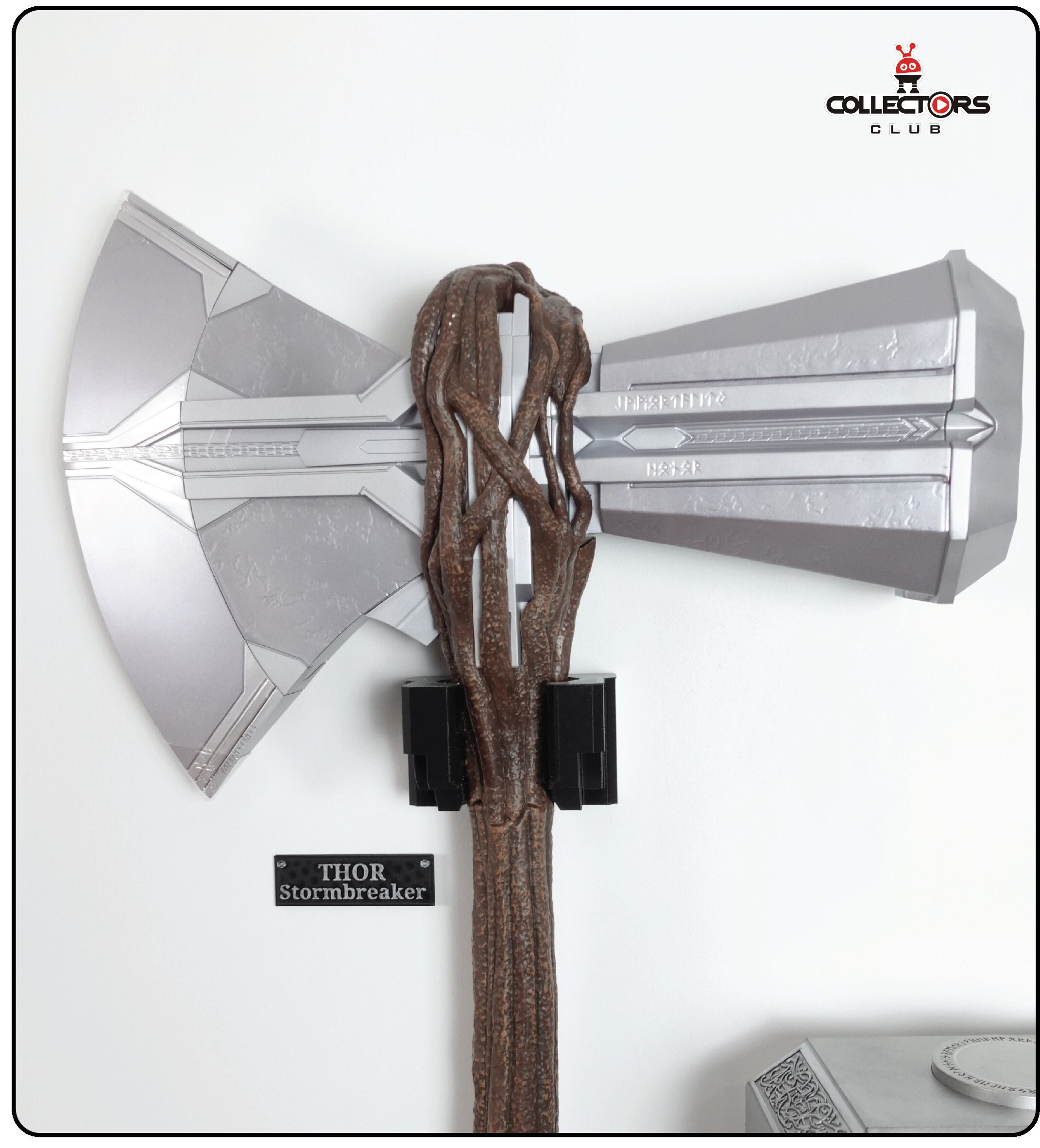The image depicts a weapon displayed against a solid white background, surrounded by a thin black border. In the upper right, there's a red and black robotic character with the inscription "Collectors Club," where the 'O' contains a play button-like logo. The focal point is the weapon identified as "Thor Stormbreaker" on a black plaque with silver lettering to its left. The weapon features a unique design: a brown, replica wooden handle made of delicate, separated strips of wood that cradle the silvery metal components. One end of the weapon forms a hammer, while the other end is an axe blade. The weapon is suspended by a black clip, and additional intricate etchings can be seen on it, adding to its detailed craftsmanship.